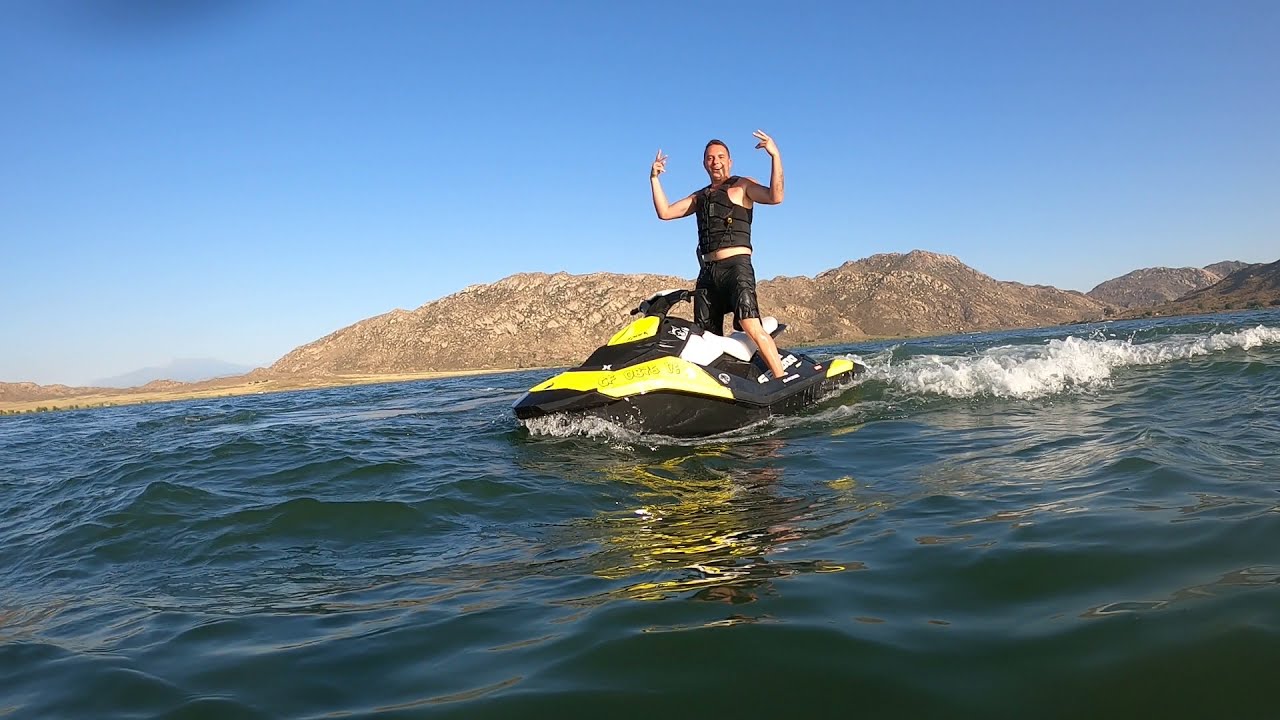This is a wide, high-definition photograph capturing a man standing triumphantly on a jet ski in what appears to be a lake or possibly an ocean. The bottom half of the image features slightly wavy, bluish-gray green water. The jet ski, black with yellow and white accents, is positioned in the center of the frame and points towards the bottom left corner. The man on the jet ski, who has white skin and short brown hair, radiates confidence as he smiles at the camera, hands raised in a peace sign. He is dressed in black shorts and a black life vest. Behind him, a line of rugged, brown and gray mountains slopes diagonally upwards, providing a dramatic backdrop against the clear, blue, cloudless sky. The water behind the jet ski churns into a white wake, adding dynamic movement to the serene landscape.